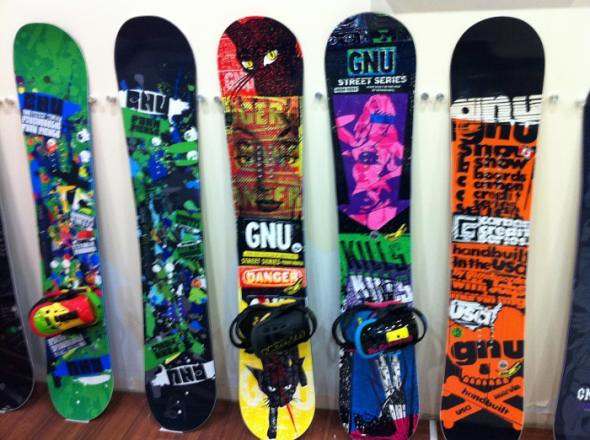The photograph depicts five snowboards leaning against a white wall on a dark brown wooden floor. From left to right:

1. The leftmost snowboard is predominantly bright green with a chaotic, graffiti-like splattering of multiple colors in the middle. It also features a red section where a foot holder might be.
   
2. Next to it is a mostly black snowboard accented with green, navy, and bright blue splatters. It has "GNU" printed multiple times and appears to have foot holders that are less visible.

3. The middle snowboard is a vibrant mix of yellow and red with black cats at the top and bottom. It has "GNU" and "DANGER" written on it, along with the image of a woman's face, resembling Marilyn Monroe, with a visually striking combination of red and black overlays.

4. To the right of the middle board is a predominantly navy snowboard with "GNU STREET SERIES" at the top. It features a patch-covered purple box with a pink go-go dancer in a blue bikini. Words like "KILLS" are written over the design.

5. The rightmost snowboard, partially cut off in the photo, has a black background with an orange design incorporating a skull and crossbones, more text including "GNU" and "USA", and a scattering of other lettering.

All five boards are positioned upright, angled against the wall, with the photo taken slightly askew so that the farther boards appear smaller.